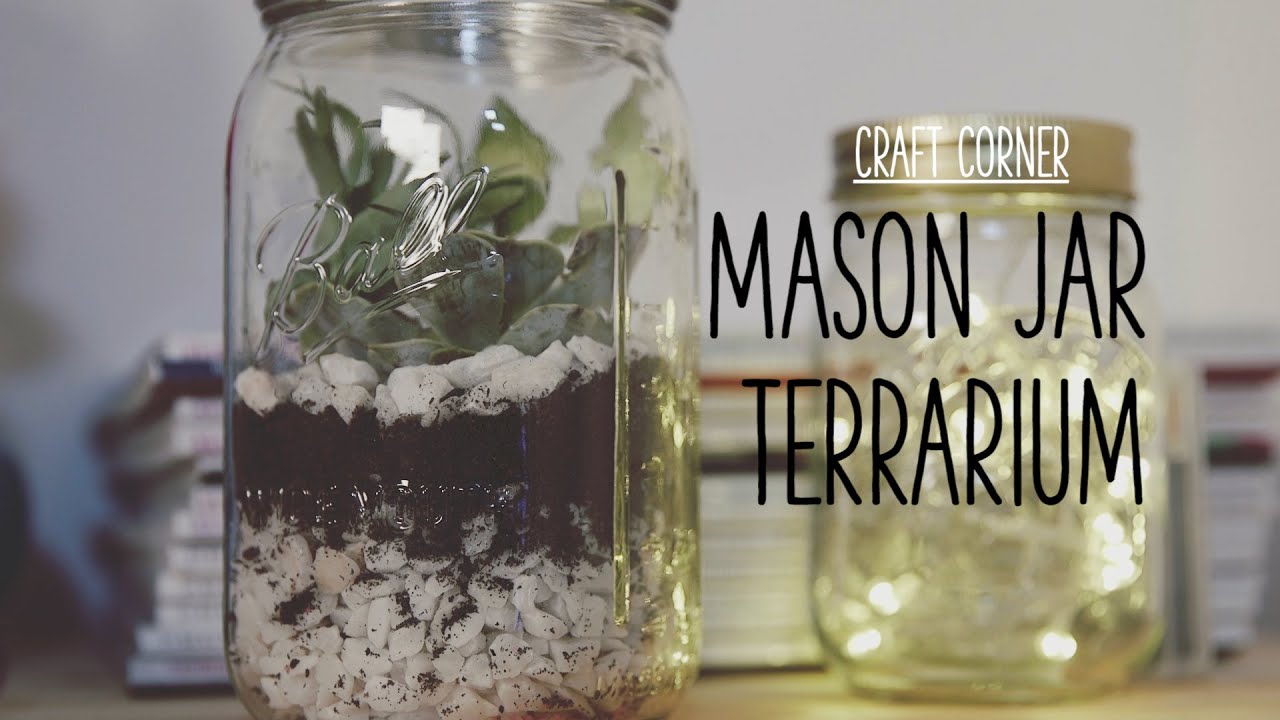This photograph showcases an enchanting scene of two mason jar terrariums placed on a wooden surface against a blurred light gray wall backdrop. In the foreground, a clear Ball glass mason jar, approximately the size of a quart, houses a meticulously layered terrarium. It starts with white stones at the bottom, followed by a layer of rich soil and topped with more white stones and lush green foliage filling the upper third of the jar. The jar is lidded and exhibits the "Ball" logo proudly on its front. 

Behind this focal terrarium, another mason jar is barely in focus. This jar features a gold cover and seems to contain a twirling line of fairy lights, which add a magical glow. To the right side of the image, superimposed text reads "Craft Corner Mason Jar Terrarium," with "Craft Corner" in underlined white text at the very top and "Mason Jar Terrarium" below it in black text. The background is softly blurred but reveals a stack of books, magazines, or posters, adding a cozy, cluttered charm to the scene.